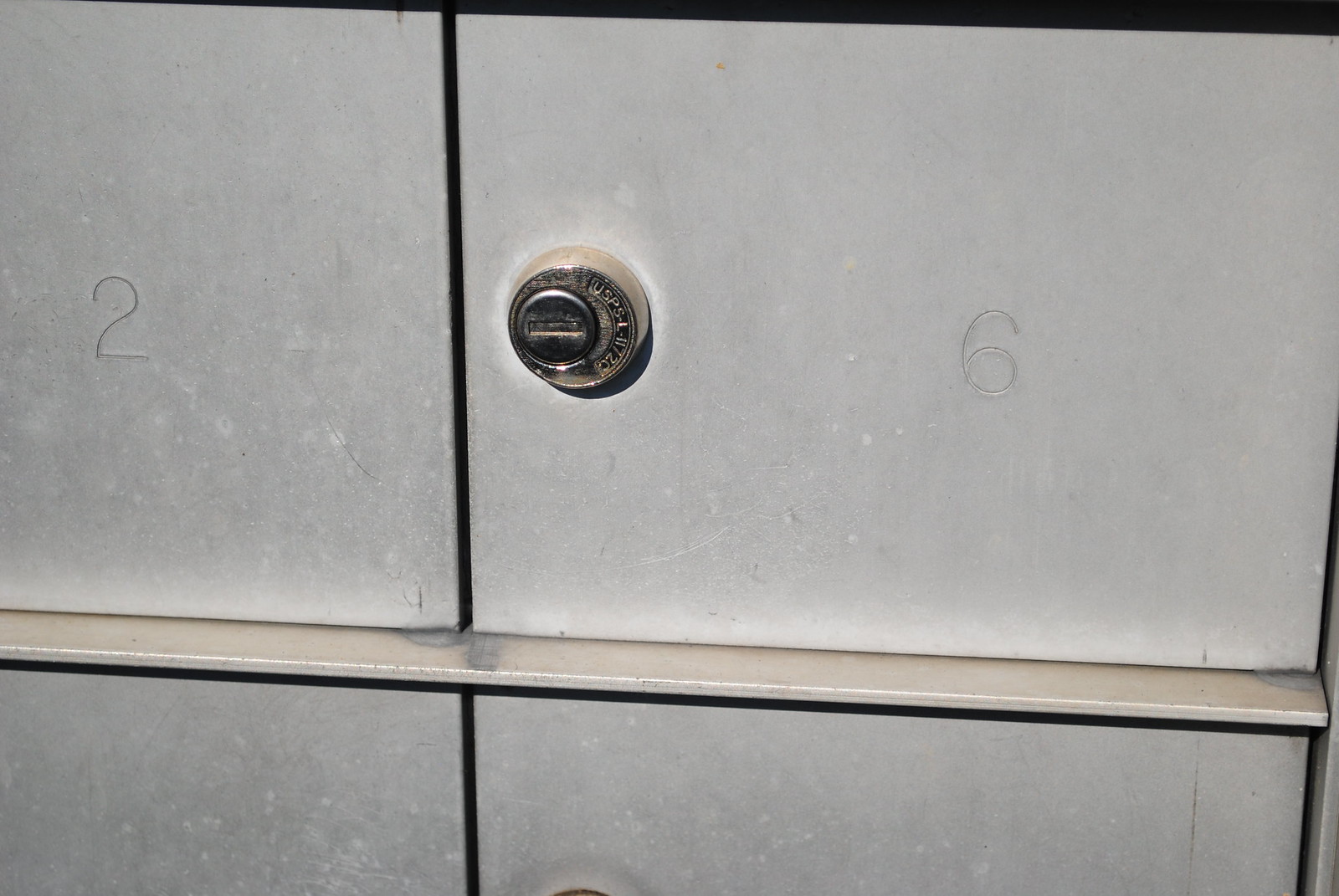This detailed color photograph captures a close-up view of several weathered and worn metal mailboxes, likely found in an apartment building. The mailboxes are arranged vertically and appear slightly rectangular rather than perfectly square, with their surfaces showing signs of scratches and dirt. A brass-colored circular lock, with an off-center keyhole, is visible prominently on the mailbox marked with the number 6, located at the top right. Another mailbox, labeled with the number 2, is faintly visible at the top left. The mailboxes are painted a tan or beige color, and partially shown, with no visible locks on the remaining units. The mailbox labeled with 6 includes the designation "USPS-L-1112C" beside its lock, indicating it is part of the U.S. Postal Service's standard locking mailbox system. The image presents a functional yet somewhat neglected look, emphasizing the everyday, utilitarian aspect of communal mailboxes.